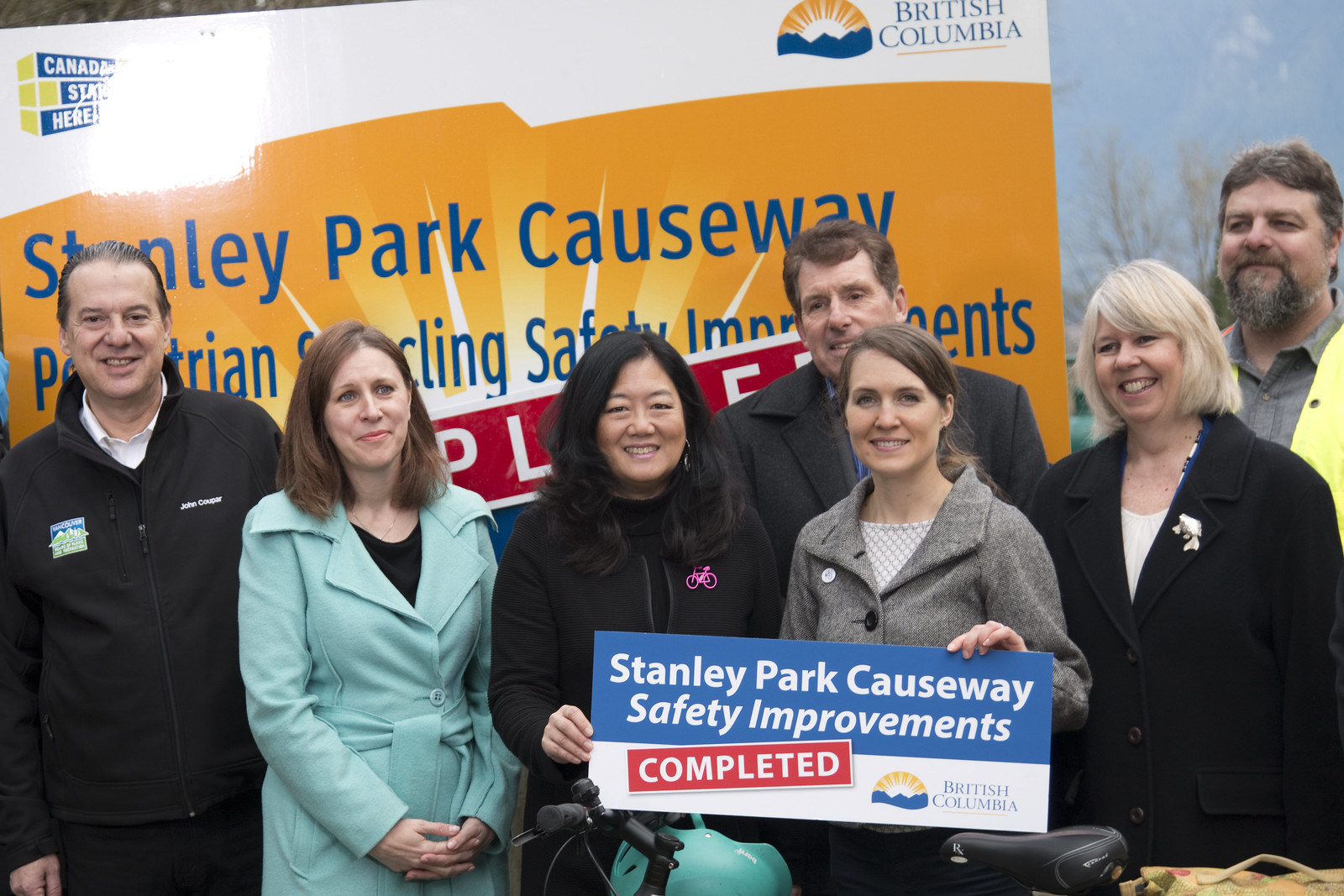This photograph captures a group of seven middle-aged men and women posing outdoors in front of a large orange billboard that prominently features the text "Stanley Park Causeway Pedestrian & Cycling Safety Improvements Completed" in white, red, and blue colors. The billboard also displays "Canada starts here" on the top left and "British Columbia" on the top right, along with a sun symbol. The group consists of four women standing in the front line, two of whom are holding a smaller sign that reiterates "Stanley Park Causeway Safety Improvements Completed." Behind them stand three men, likely all part of the team responsible for the project’s completion. The individuals are mostly dressed in dark colors, except for one woman in a light blue coat and another in a gray coat, and they are all smiling proudly at the camera. A bike can be seen in the foreground, symbolizing the emphasis on pedestrian and cycling safety improvements being celebrated.